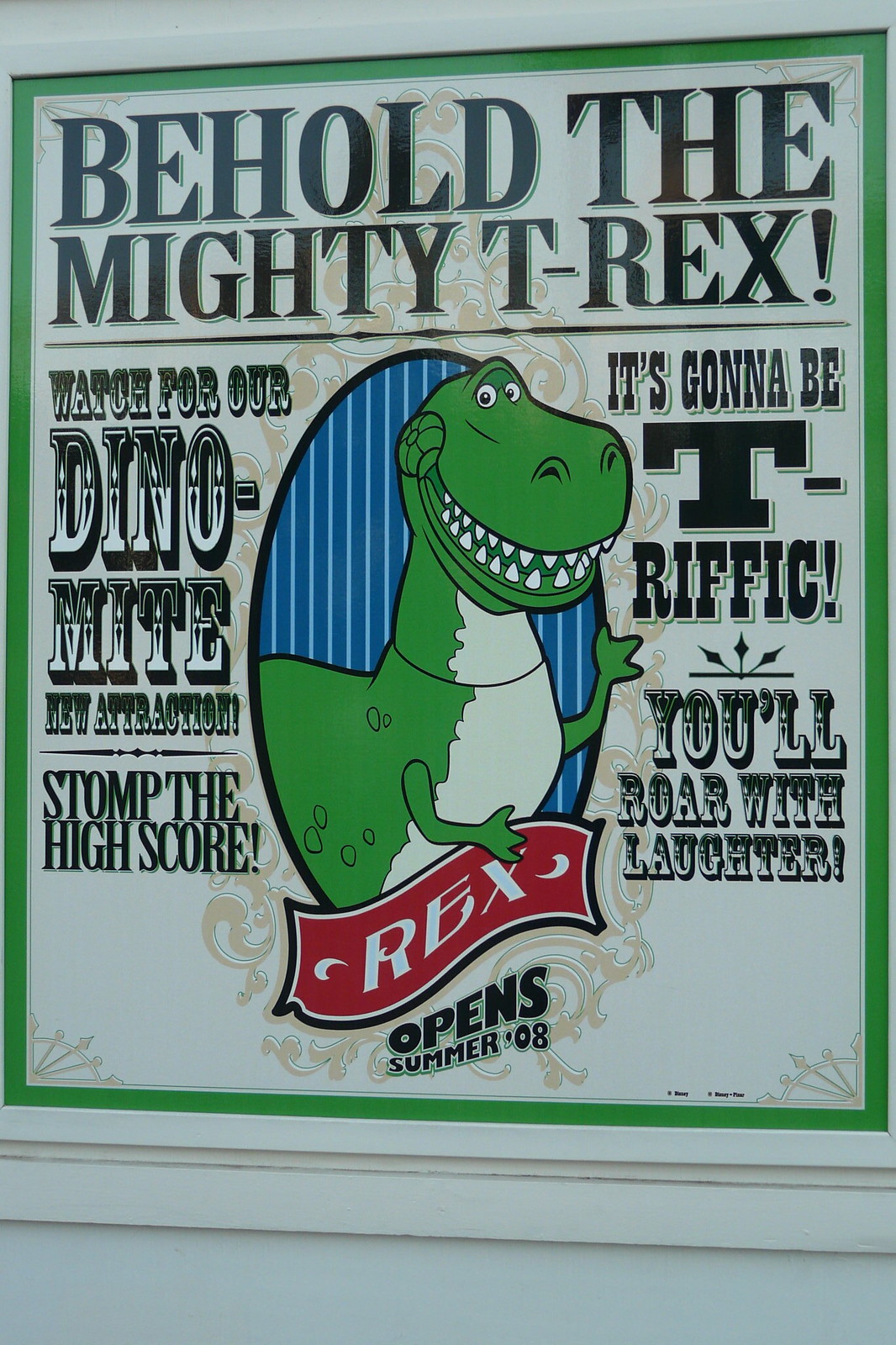The image features a vibrant sign with a green border that promotes an upcoming attraction. Dominating the center is a cartoonish drawing of the green T-Rex, Rex, from Toy Story, depicted smiling within a blue oval with white stripes, almost like a mirror. The top of the sign boldly announces in black text, "Behold the mighty T-Rex!" To the left, additional text teases, "Watch for our dino-mite new attraction," followed by "Stomp the high score." On the right, it reads, "It's gonna be T-rific," and underneath that, "You'll roar with laughter." Beneath the cheerful T-Rex is a red ticket-like banner with "Rex" in white text and below it, in black text, "Opens summer '08," hinting at a new, exciting offering, potentially at an amusement park or involving a video game challenge.